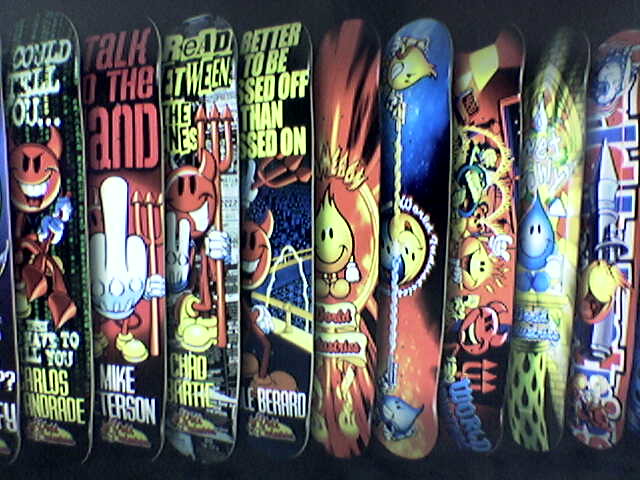The photograph showcases a highly colorful and detailed arrangement of nine skateboard decks, artistically displayed against a plain black background. Each deck is angled and slightly overlapping, emphasizing their vibrant designs. On the far left, a heavily cropped skateboard end is barely visible. Prominent on these decks are recurring motifs and characters, hinting at a cohesive artistic style likely from a single artist or company. Central to the designs are devilish and mischievous characters: a red devil orb frequently flipping the viewer off and holding a pitchfork appears multiple times, along with another red devilish smiley face. Additionally, there are playful flame characters - one yellow with a tuft of hair, more smiley and easygoing, and a blue raindrop-like figure. In one scene, a yellow and a blue flame character are depicted in an intense standoff, shooting colorful beams at each other. The color palette is dominated by reds, blacks, yellows, whites, and blues, with occasional greens on the far-left deck. These decks, devoid of wheels, provide a dynamic and striking visual presentation, likely intended for promotional use.